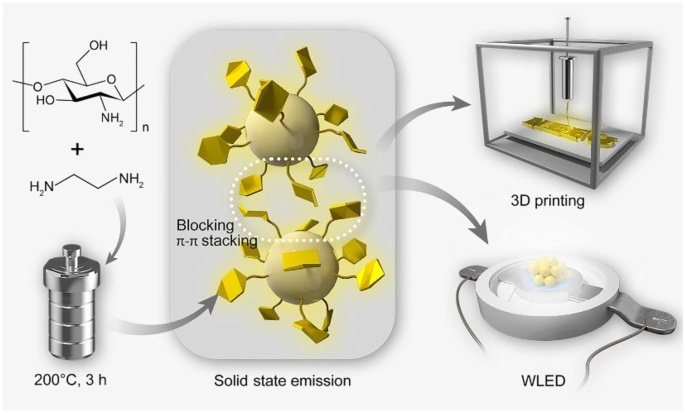This detailed diagram, typically found in textbooks or scientific papers, provides a comprehensive illustration of molecular structures and their applications. On the left, it showcases intricate, non-linear graphs depicting chemical compounds with labels of OH, O, and NH2 in various arrangements. Below these graphs, a metallic cylinder is prominently displayed, with a caption beneath it reading "200 degrees Celsius, 3 hours." 

Centrally positioned, the diagram highlights two rounded spheres with yellow hexagons and rectangles emanating from them, illustrating the concept of blocking pi-pi stacking. This section is captioned "solid state emission," emphasizing the interaction of these molecular structures.

Moving to the right, the illustration transitions into technological applications. A glass box symbolizes a 3D printer, and positioned below, there is a circular object equipped with twin metallic components on its sides, labeled "WLED." This part highlights the practical implementation of the chemical processes depicted, rounding out the scientific narrative presented in the diagram. The entire illustration is set against a white background, with colors primarily from the molecular illustrations and textual annotations, enhancing the visual appeal and clarity of the scientific concepts being conveyed.